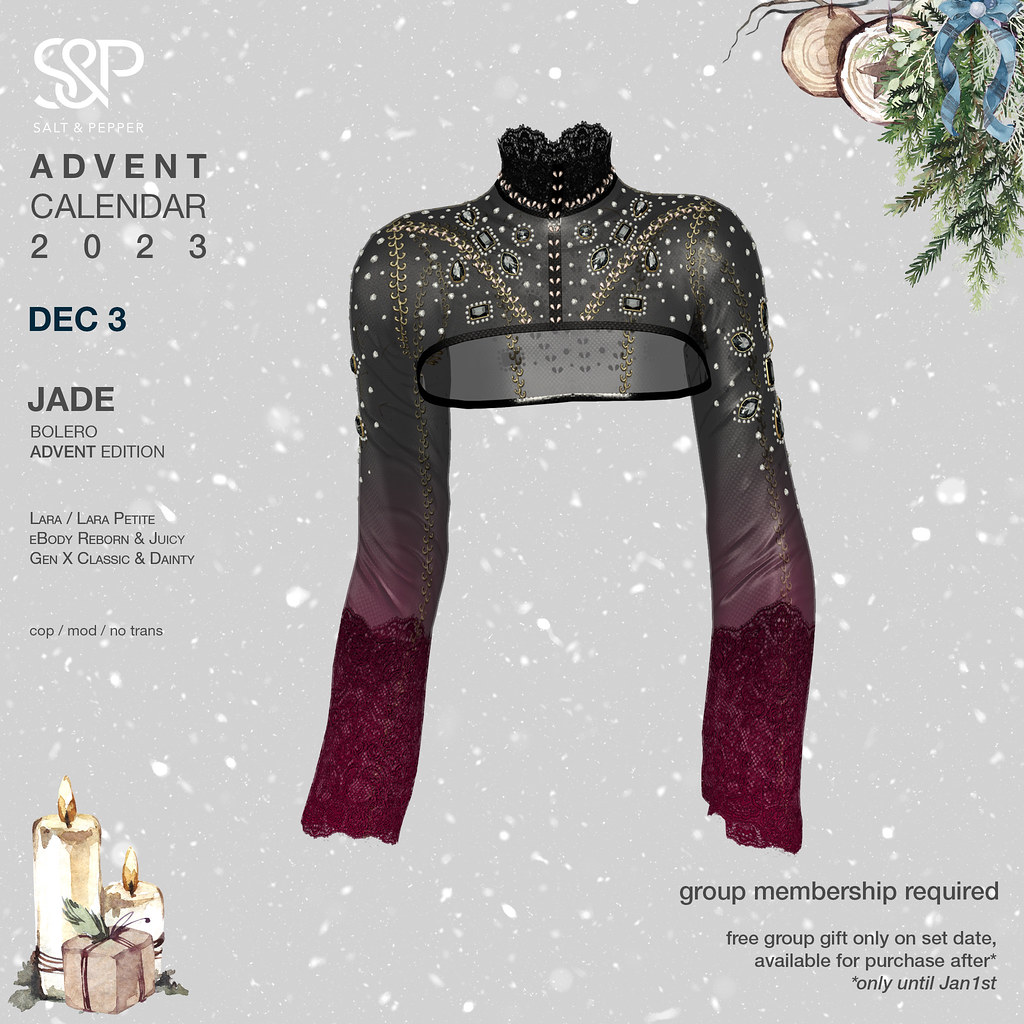**Caption:**

The image showcases a stylish, loose-fit top resembling a bolero. This garment is designed to cover the upper part of the abdomen and features intricate decorative designs highlighted with subtle light jewels. The color palette of the top transitions from a soft gray at the top to a vibrant red at the bottom. On the left side of the image, the text reads "S&P Advent Calendar 2023 December 3" followed by "Jade Bolero Advent Edition." Below this text, smaller, unreadable words are displayed. The bottom left corner features a whimsical illustration of candles and a gift box, while the bottom right corner includes the message: "Group membership required, free group gift only on set date, available for purchase after only until January 1st." In the top right corner, a sprig of mistletoe adds a festive touch to the advertisement.